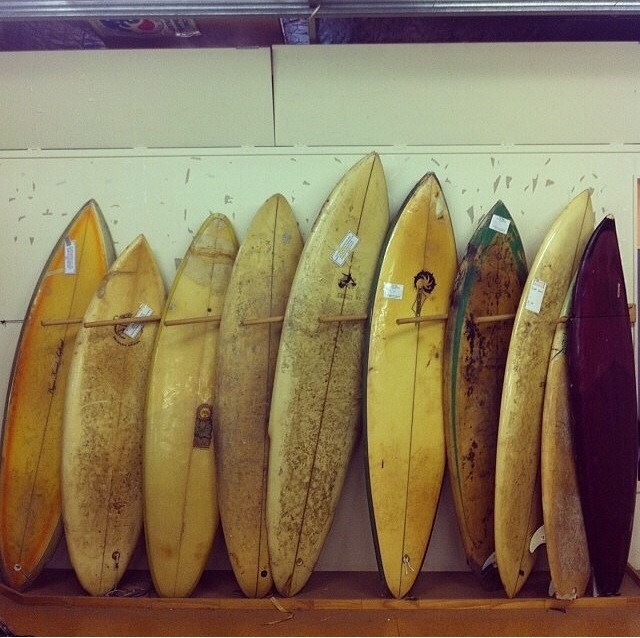This photograph captures a somewhat dimly-lit storage area or possibly a shop, where a collection of approximately ten to thirteen surfboards is neatly organized. The surfboards, which are clearly worn and weathered from use, stand upright, leaning against a white wall, held in place by wooden pegs protruding from the wall. Most of the boards exhibit various shades of yellow, with several displaying a pale yellow hue and a few brighter ones. A couple of the surfboards deviate from this palette, with at least one appearing dark brown and another with some green paint in the middle. Interestingly, there are white tags visible on several of the boards, suggesting they might be for sale or awaiting repair. The surfboards have a mix of finishes, some looking like tan wood, while others seem to have a more artificial, distressed aesthetic. The background wall is somewhat scuffed, further emphasizing the rustic and well-used nature of the place.